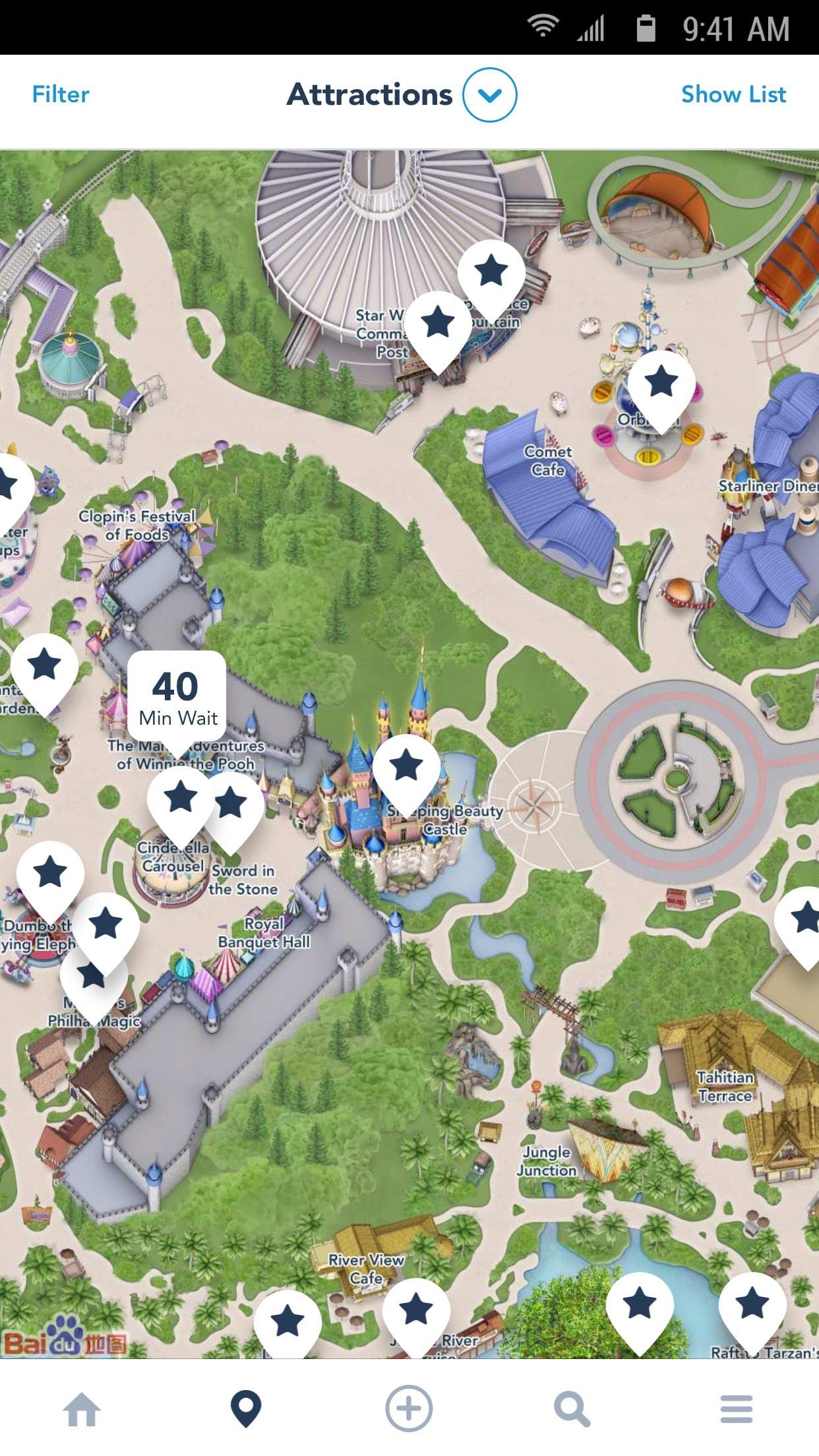This image appears to be a screenshot from a mobile app, likely displayed on an Android device, based on the recognizable icons and layout. The top of the screen shows a black status bar with the time set at 9:41 AM, a battery life approximately between 70-80%, and strong signal strength for both Wi-Fi and cellular networks.

Below the status bar, there is a white navigational strip. On the left in blue text is the word "Filter," and on the right in blue is "Show List." Centered between these is the word "Attractions," accompanied by a circular button with an arrow, suggesting that users can click it to view a list of attractions.

The main portion of the screen is occupied by a cartoony, overhead map of what appears to be an amusement park or zoo. The map is detailed with buildings, green spaces, and trees. Various attractions are highlighted with call-outs containing stars and text indicating features or wait times. Some notable attractions include:

- A 40-minute wait near the "Magical Adventures of Winnie the Pooh"
- "Cinderella Carousel"
- "Sword in the Stone"
- "Royal Banquet Hall"
- "Dumbo the Flying Elephant"
- "Clopin's Festival of Food"
- "Comet Cafe"
- "Starliner Diner"
- "Star Wars"
- "Tahitian Terrace"
- "Jungle Junction"
- "Riverview Cafe"

At the very bottom left corner, there is a logo with the letters "BAI," a graphic of an animal paw with four toes, the letters "DU," and some Chinese characters, suggesting a connection to Baidu, a well-known Chinese search engine and technology company. This detail, combined with the inclusion of Chinese characters, indicates that the app might be affiliated with Baidu or developed for a Chinese-speaking audience.

Considering the blend of both international and familiar Disney-themed attractions, it is plausible that the map is of a Disney park located in China, possibly Shanghai Disneyland or Hong Kong Disneyland. Overall, the mixture of known and less familiar elements points to an elaborate and immersive theme park experience.